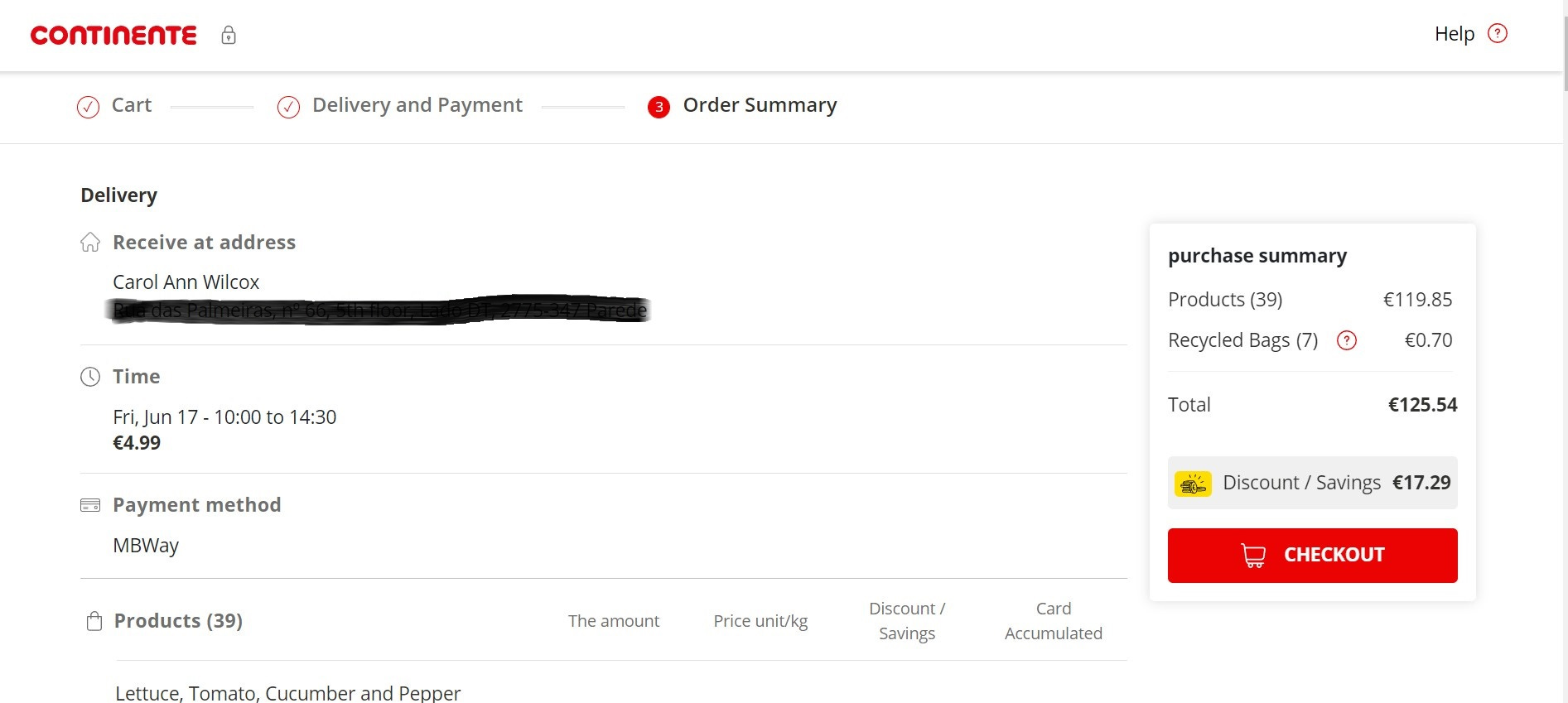The screenshot captures a segment of an online shopping interface from the website or app "Continente." At the top, progress indicators show that the "Cart" and "Delivery" steps have been completed, and the user is currently at the "Order Summary" stage, marked as step three.

On the left side under a house icon, there's a section titled "Delivery." It states that the delivery will be received at the address belonging to Carol Ann Cox Wilcox, though the specific address details have been obscured. Below this, a clock icon indicates the delivery time, scheduled for Friday, June 17th, between 10:00 AM and 2:30 PM, with a delivery fee of 4.99 euros. The payment method chosen is MB WAY.

The order summary lists 39 products with a subtotal of 119.85 euros, plus an additional 0.70 euros for recycled bags, bringing the total to 125.54 euros, highlighted in bold. There is also a highlighted discount savings of 17.29 euros.

Towards the bottom, a prominent red button with a white shopping cart icon prompts the user to "Check Out." Adjacent to this, in a section summarizing the 39 products, details such as unit prices, discount savings, and cart accumulation are provided. The visible items include lettuce, tomato, cucumber, and pepper, but the full list of purchased items is cut off in the screenshot.